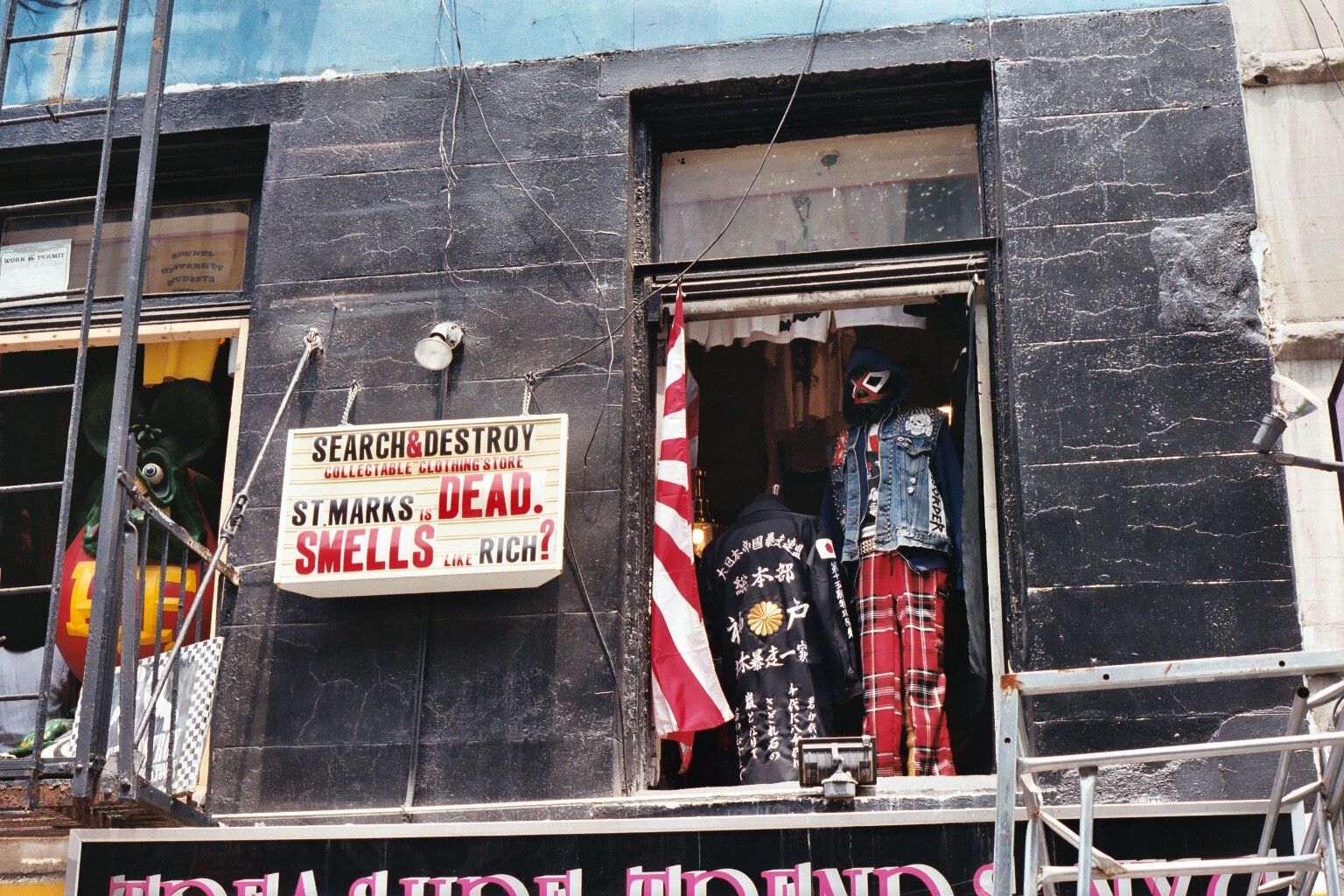This photograph captures a second-story shop window of a dark gray, slightly grungy building. The image is taken from the ground, looking up, revealing a vivid display in the window. One mannequin, adorned in a denim jacket and red plaid pants, possibly pajama-style, is partially turned towards the viewer and even wears a mask. Adjacent to this figure stands another mannequin, or perhaps a person, facing away from the window and draped in a long black coat featuring Chinese script and a gold emblem. To the left side of the window, hanging on the black brick facade of the building, is an elaborate sign that reads, "Search and Destroy Collectible Clothing Store." The ampersand is red while the rest of the main text is black. Below, in mixed red, and black text, it states, "St. Mark's is dead. Smells like rich?" All of this is displayed on a white announcement board, accompanied by a ladder running up the left side of the building, adding to the eclectic and slightly mysterious aura of the scene.